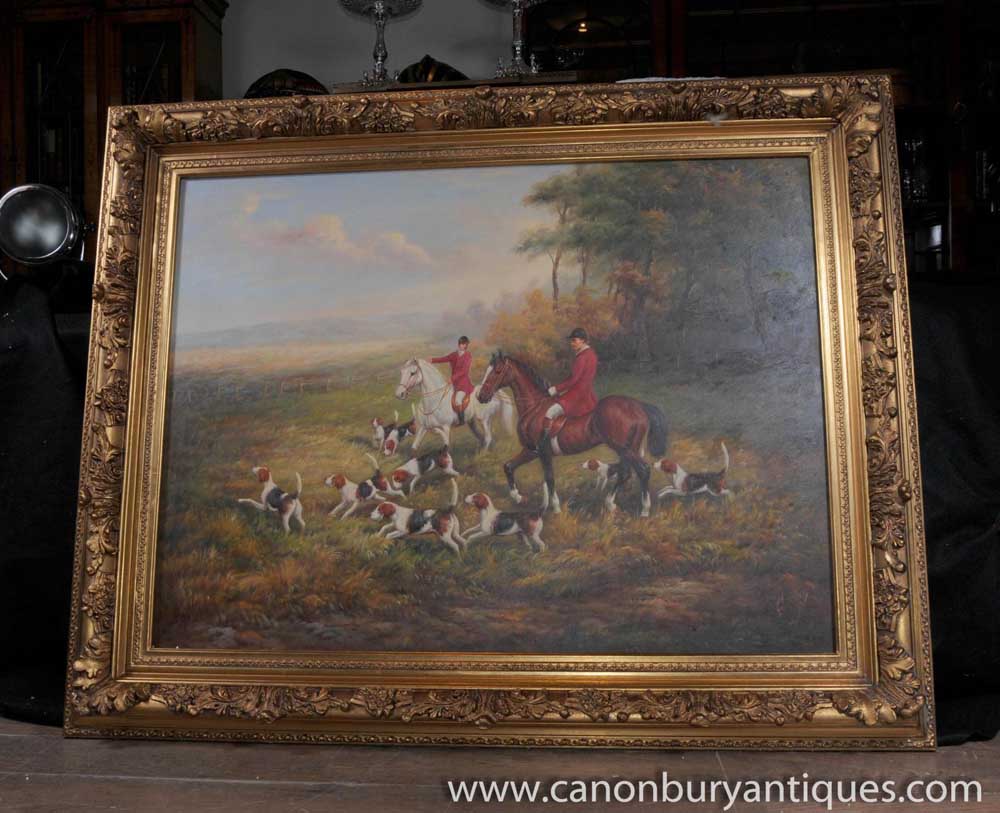The photograph captures an ornate, gold-framed oil painting depicting a vibrant fox hunt scene. The painting features two individuals clad in red jackets, white pants, black boots, and hats. They are mounted on horses, with the closer horse being brown with a black mane and tail, and the farther one entirely white. Surrounding them, a lively pack of hound dogs in shades of white, black, and brown frolic through a grassy meadow. The backdrop showcases a serene landscape with a forested area on the right and a blue sky embellished with a few clouds, suggesting a sunny day with soft, early morning or late afternoon light. The gold frame is richly decorated, with a darker gold on the outer edge and a lighter gold edging inside. The watermark "www.cannonburyantiques.com" is visible at the bottom-right corner of the image.